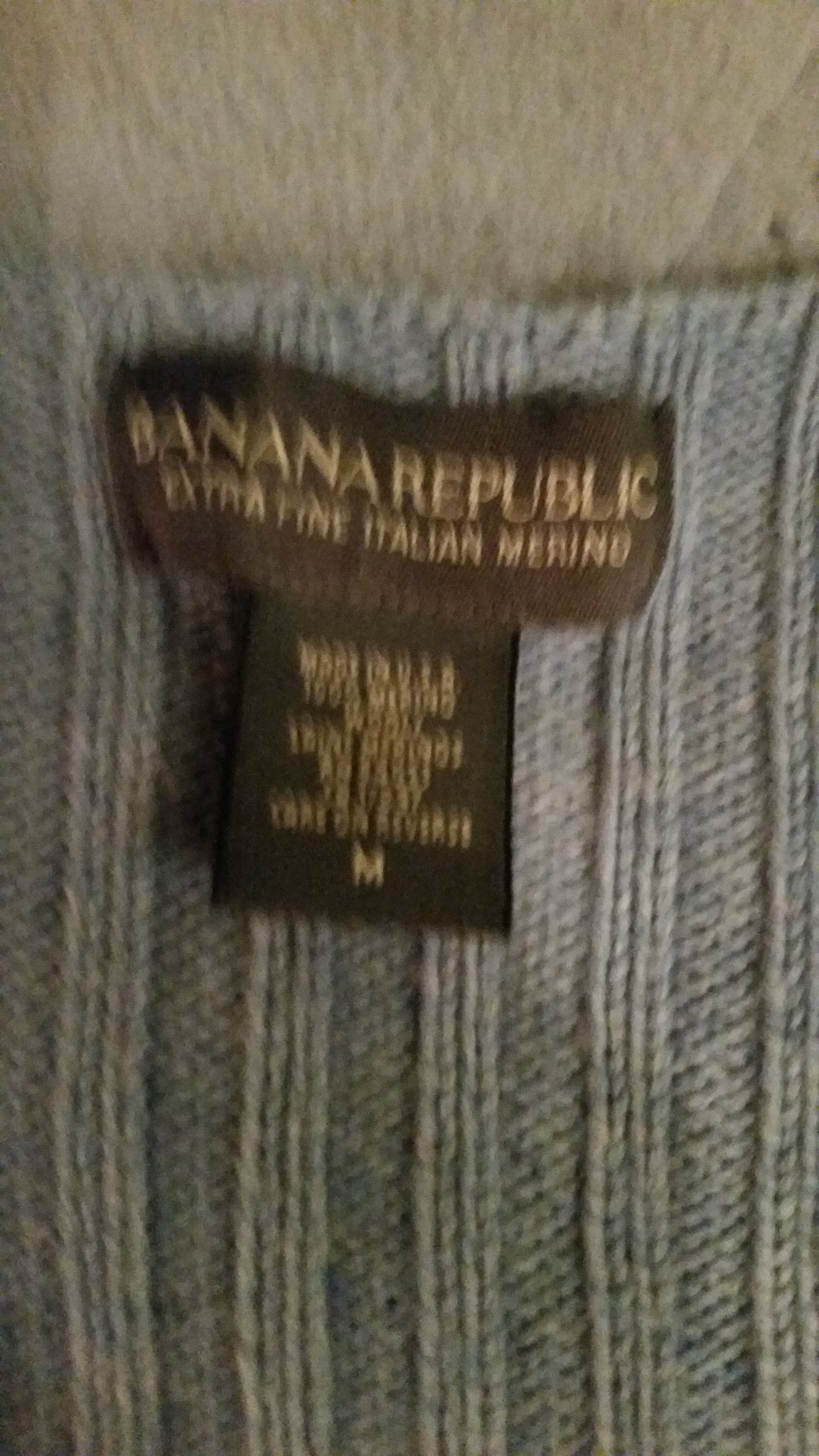A detailed, cleaned-up caption for the given image might be:

"This is a color photograph oriented vertically, capturing a close-up view of the label on a gray, vertically ribbed knit sweater. The sweater features an alternating texture with four lines of ribbing followed by four lines of regular knit, giving it a very tactile, rich appearance. The background appears to be a piece of cloth or possibly a blanket, though it is out of focus. The sweater itself stands out clearly against this blurred backdrop, enhancing the texture of its knit. The label, however, is blurry but identifiable; it is a brown tag reading 'Banana Republic Extra-Fine Italian Merino,' indicating the sweater is made of merino wool. Below this, there is another smaller, square brown tag with care instructions. Although the instructions are illegible, there is an 'M' indicating the sweater is a medium size and a note suggesting to check the reverse side for care instructions."